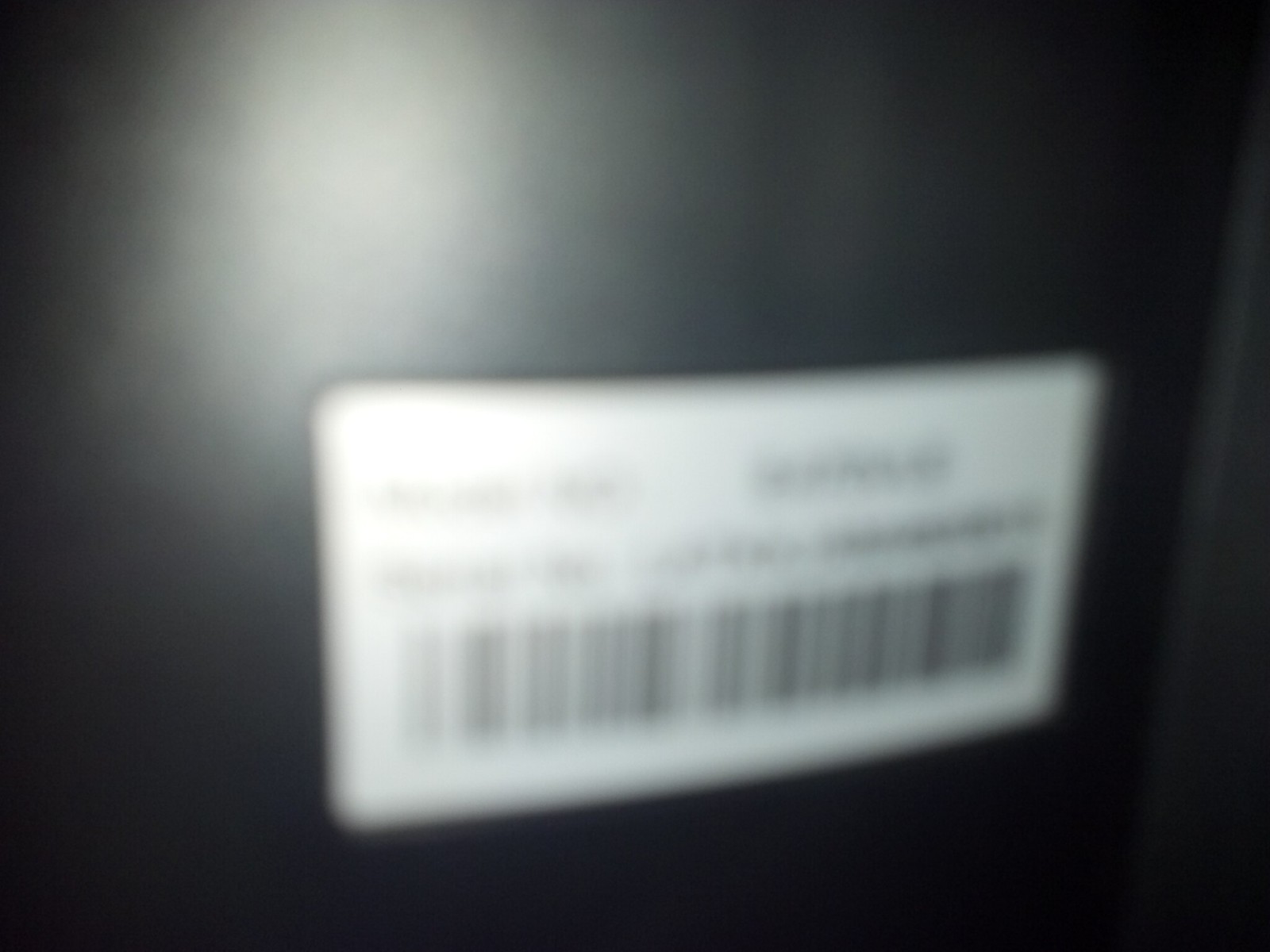This indoor photograph captures a black object prominently featuring a white rectangular label with various text elements. The label includes four lines of black writing, but due to extreme out-of-focus conditions, the letters are indiscernible. Below the text lines is a black barcode, adding a layer of utilitarian detail to the label. Part of the black object reflects a bright white light, likely caused by the camera flash. The overall image remains blurred, emphasizing the out-of-focus effect and creating an enigmatic atmosphere around the purpose and identity of the black object.